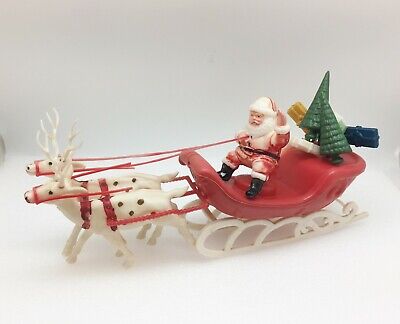The photograph showcases a vintage-style Christmas ornament against a white background. The centerpiece is a traditional ceramic Santa Claus sleigh, characterized by its vibrant red color and white sled rails. Santa Claus, donned in his classic red and white outfit, is seated in the sleigh, joyfully waving with his left arm while holding the reins in his right hand. In front of the sleigh, two white reindeer with black spots and red reins are positioned, moving from right to left. The reindeer are adorned with white antlers and are connected to the sleigh with red harnesses. Behind Santa, the sleigh features two triangular Christmas trees and a few presents peeking out from either side, in colors of gold, white, and blue. The ornament rests on a white surface, complemented by a light gray or off-white backdrop, giving a nostalgic ambiance reminiscent of past decades. The overall appearance of Santa and the sleigh indicates a charming, worn vintage aesthetic, adding to the festive charm of the scene.